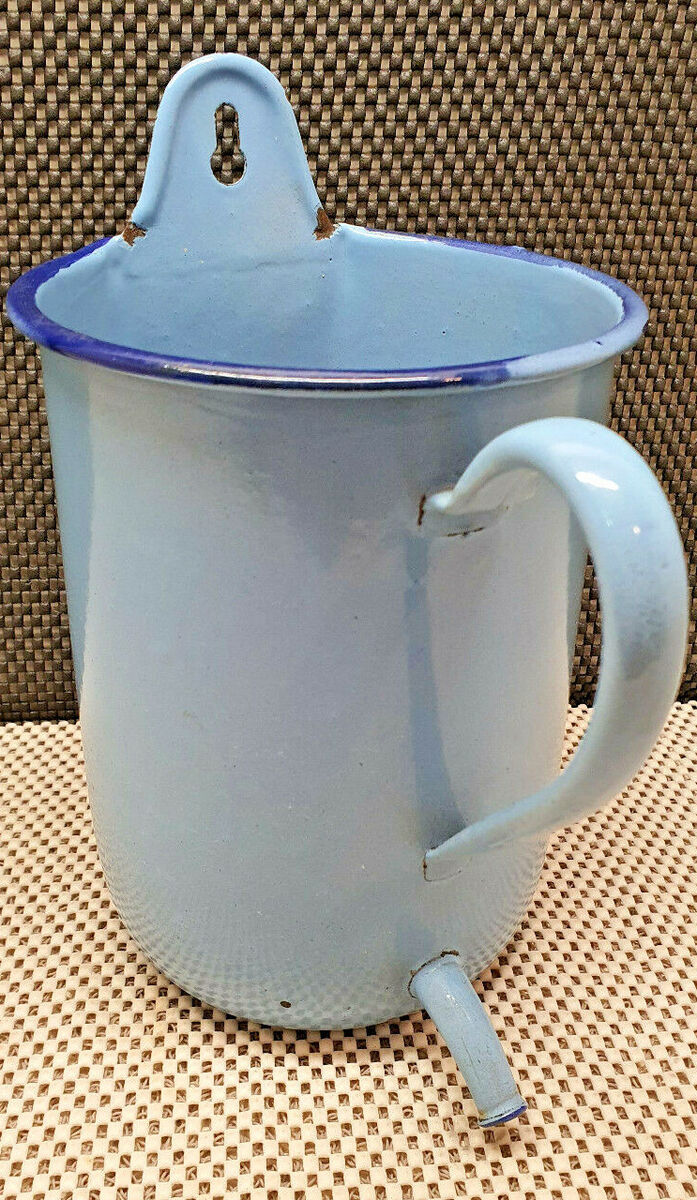The image showcases a metal-looking, antique white vessel, which could be a specialized mug or cup, featuring a unique design. The vessel has a prominent blue-bordered rim at the top, although some color has rubbed off, creating a partially blue effect. At the top rim, there's a distinctive key-shaped cutout. The vessel also has a large white handle with visible cracks and a small spout extending from the front. The vessel is set against a wicker-like background: the darker brown and golden hues behind it contrast with the light beige mat featuring small cut-out squares below it. Shadows are subtly cast on the left and center of the vessel, enhancing its depth.